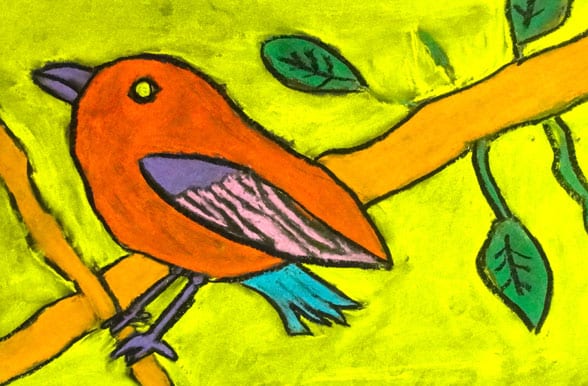This image depicts a crude, beginner's oil pastel-style drawing of a small red finch perched on a branch. The background is primarily white with areas of bright yellow and light grey, giving it a textured, almost chalk-like appearance. The main branch is a plain, narrow brown rectangle extending diagonally across the image, adorned with four small green leaves. In the left corner, another branch appears vertically and diagonally, supporting the bird.

The finch itself is drawn with beginner-like simplicity, showcasing a red body, a yellow eye encircled in black, and a slightly curved purple beak. The bird's wings feature a combination of purple and stripes in dark brown with hints of pink, and possibly a light blue or teal at the tail. The bird's legs and feet are depicted in purple, adding to the colorful yet unrefined charm of the artwork.